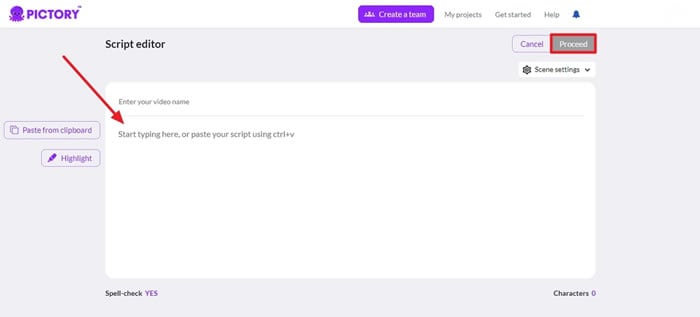This image captures a screenshot from a computer display, showcasing the Pictory website interface. Prominently featured is a character resembling a purple octopus, adjacent to which the word "PICTORY" is displayed in bold, purple text. 

Across the top navigation bar are various options: "Create a Team," "My Projects," "Get Started," and "Help," where a blue bell icon is situated. The background of the webpage is a large gray rectangle, with a white rectangle nested inside it.

At the top of the white rectangle, the title "Script Editor" is visible. A red arrow is highlighted on the left side of the screen, pointing towards the text box labeled "Start typing here or paste your script using Ctrl + B."

Additionally, towards the top of the screen, the word "Cancel" is written in purple. Directly next to it, "Proceed" is displayed within a gray rectangle, which is now outlined by a red line.